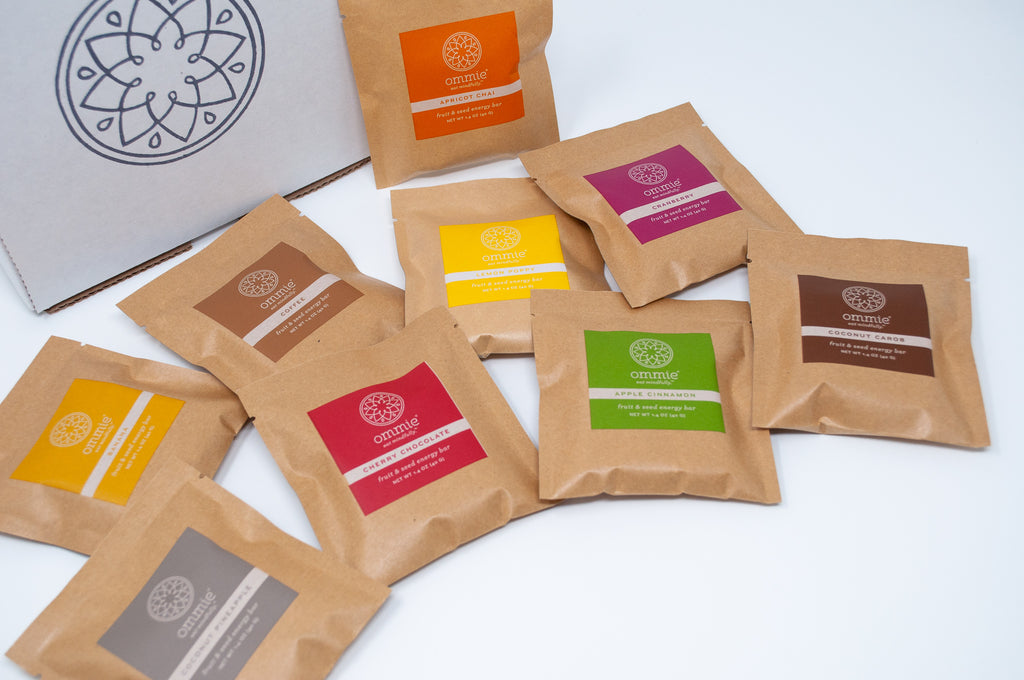Displayed on a white tabletop are nine brown paper packets, each adorned with a distinctive colored label indicating various flavors. These packets feature a circular logo with the name "OMMIE". Inside, they contain energy bars in flavors such as cherry chocolate, coconut pineapple, coffee, banana, lemon poppy, cranberry, apple cinnamon, and apricot. Each label is color-coded, with labels including gray, dark yellow, brown, dark red, bright yellow, green, purple, black, and orange. Behind the neatly fanned-out packets is a white box featuring a floral logo, tying the display together.